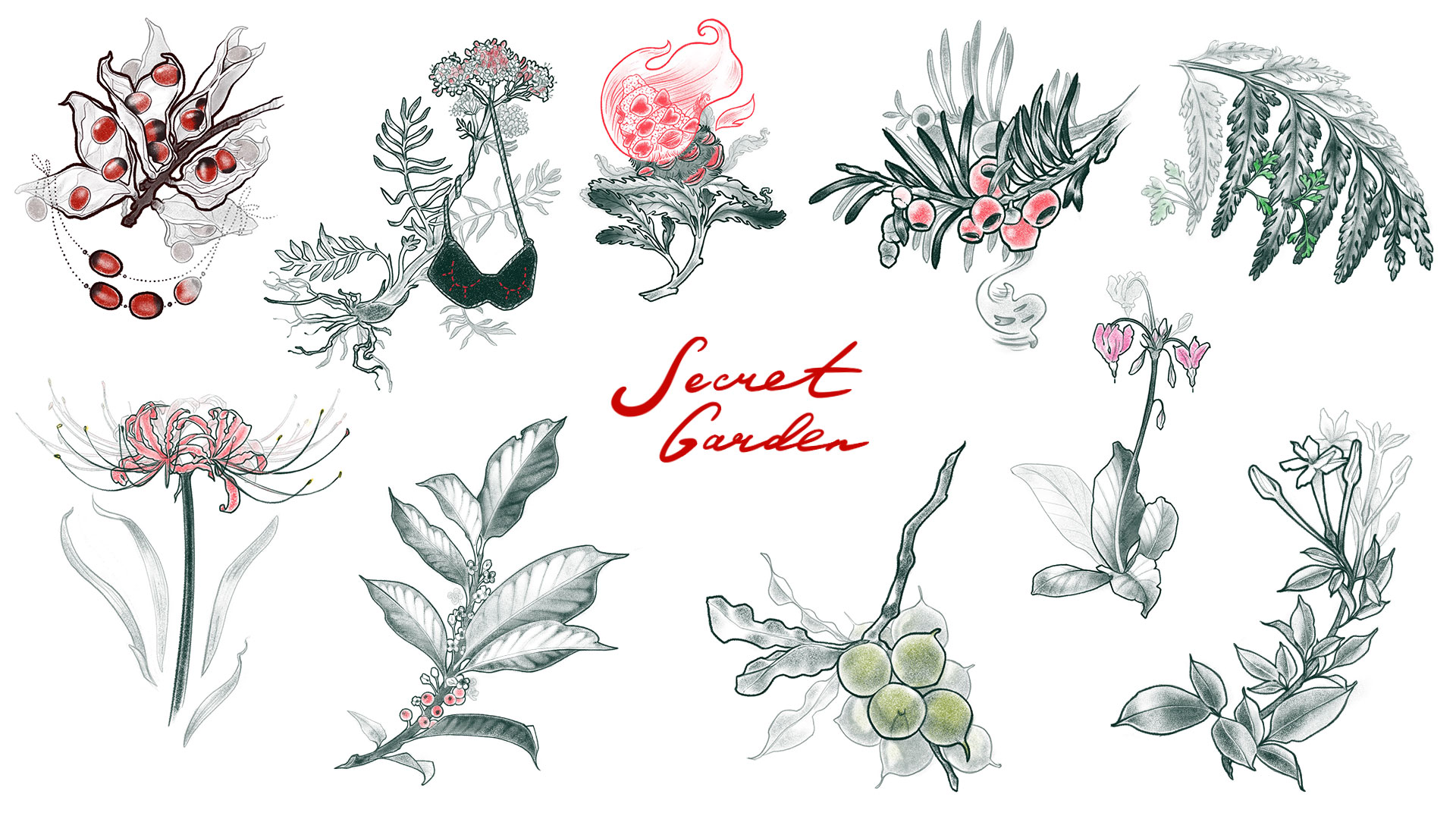This image is a detailed pencil drawing of various plants and flowers, with the text "secret garden" written in cursive red ink at the center. The drawing is organized into two rows with five distinct plant sketches each. Many plants feature greenish-white leaves, lightly colored, and the use of subtle shading. 

In the top row, there's a plant with red berries, another resembling a pine tree with pine cones, and a sketch featuring heart-shaped flowers alongside a red flame. One plant appears to have a bra tied to it, introducing a quirky detail, and another showcases red fruits. The bottom row includes a variety of plants: one with lime-colored fruits, a rose-colored petal flower, some with jagged green leaves, and others featuring pink, violet, and various shaded flowers.

The plants are delicately hand-drawn, capturing the intricate details of leaves, twigs, and branches. Some elements include a hint of color, like the pink petals and green stems, enhancing the pencil sketches' natural beauty. The composition and the "secret garden" inscription in red ink give the drawing a whimsical, enchanting feel.